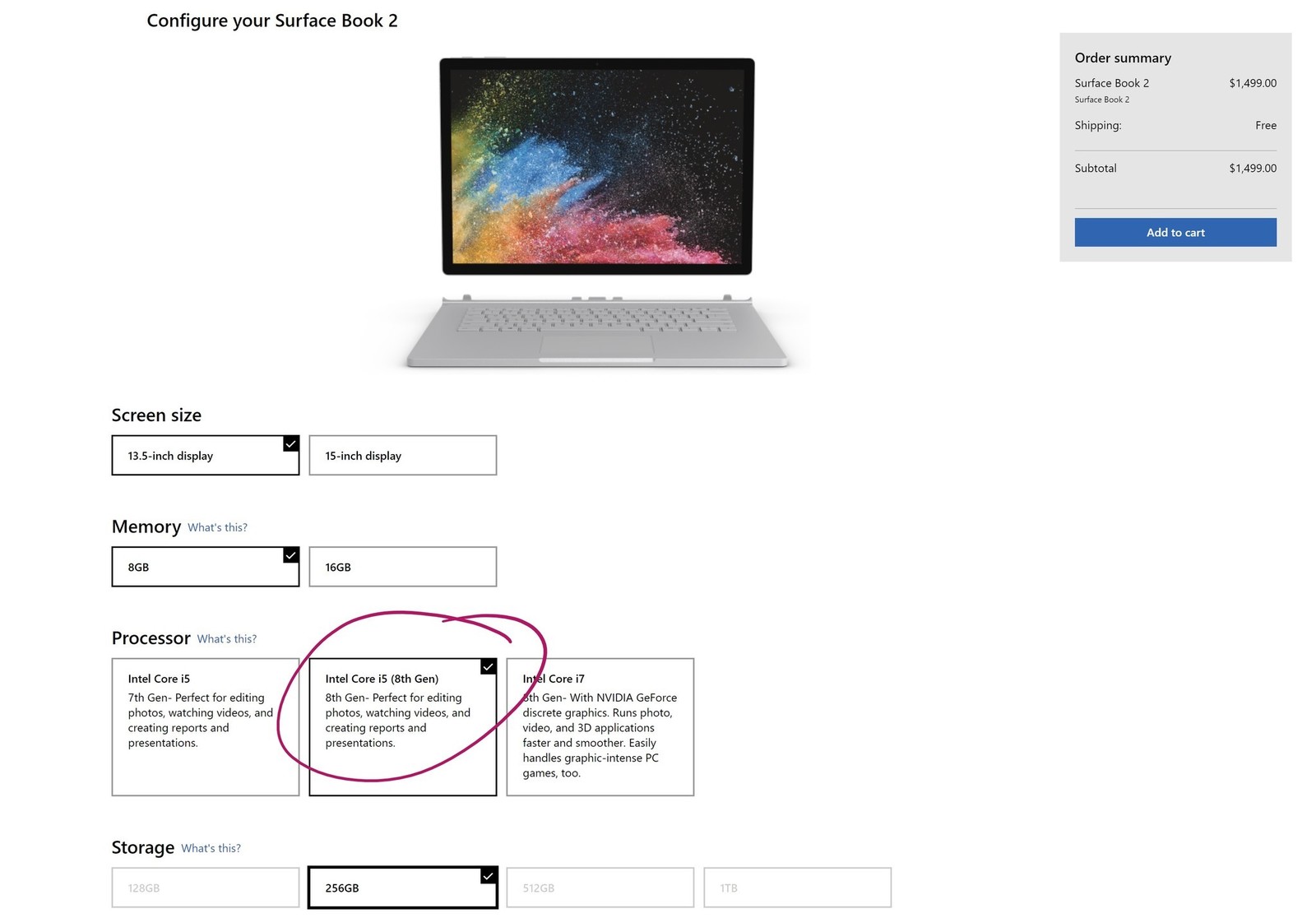Description: The image displays a customization page for the Surface Book 2 against a white background. At the top, in black font, it reads "Configure Surface Book 2." The Surface Book 2 is depicted with its screen detached from the keyboard, showing the keyboard below. The keyboard lacks a number pad and features keys spanning from Esc to the left arrow key, along with a trackpad, all in a monochrome gray color scheme.

The customizations presented in the image include options for screen size, memory, processor, and storage. The screen size options show a selected 13.5-inch display (outlined in black) and an unselected 15-inch display (outlined in gray). For memory, 8GB is selected (with a black outline and check mark), and 16GB is not selected (outlined in gray). There's also a blue "What's this?" link for more information about memory options.

The processor section shows the Intel Core i5 8th generation option as selected (highlighted with a purple circle), indicating someone's preference or recommendation. Storage options include 128GB, 256GB (selected), 512GB, and 1TB, with only the 256GB option outlined in black indicating selection. The other storage options are outlined in gray.

Above the customization options, there is a gray order summary panel. The order summary lists the Surface Book 2 at a price of $1,499, with free shipping, making the subtotal $1,499. At the bottom of this panel, there is a blue "Add to Cart" button.